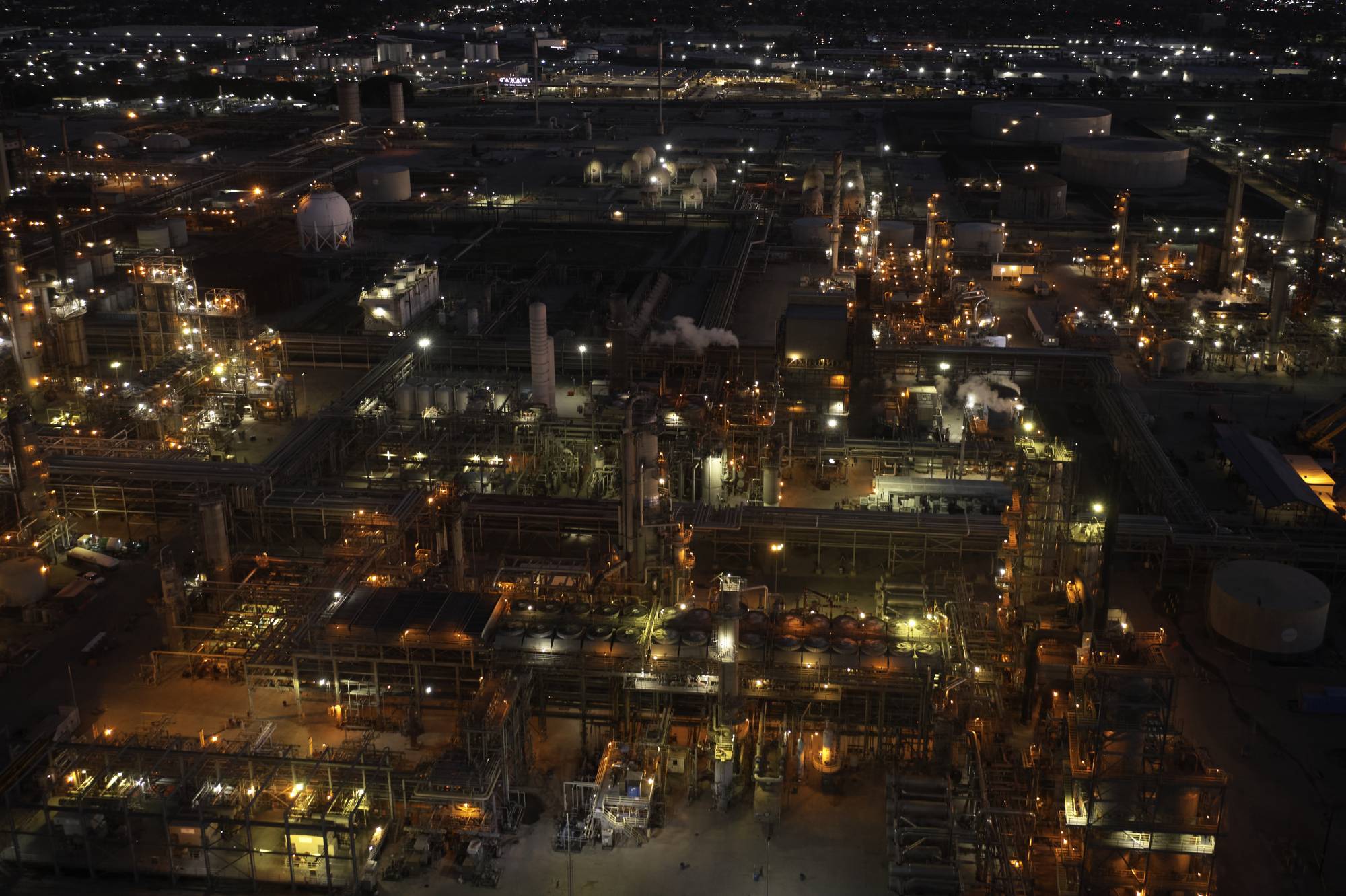The nighttime aerial photograph captures a large industrial factory with a cityscape in the background. The rectangular image, measuring approximately six inches wide by four inches high, showcases a factory complex marked by an intricate network of metal pipes, cylindrical storage buildings or domes, and numerous smokestacks. While some smokestacks emit smoke, others remain inactive. The upper portion of the photograph, about half an inch down from the top corners, reveals a dimly lit city skyline adorned with scattered lights, further accentuating the factory’s isolated appearance. The factory itself is illuminated by a mix of yellow and white lights, casting a warm glow across the scene and contributing to an overall grayish-yellow hue. Despite the inviting illumination, the factory seems deserted, likely taken after working hours, emphasizing the absence of visible workers and the tranquility of the night.